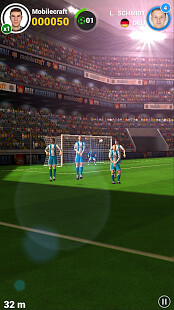This detailed caption combines the shared elements and specific details from each description to provide a comprehensive view:

"This is a screenshot from a soccer video game. The main focus is the stadium, filled with a cheering crowd, and a running track that separates the audience from the field. On the field, there are three soccer players standing in the middle, facing the viewer, with a goalie visible in front of the goal in the background. The representation is flat, typical of a video game screen.

At the top of the screen, there is an icon featuring a white man’s face within a circle, labeled ‘MobileCraft.’ Next to his image, it indicates he has accrued 50 points and a multiplier of times 1. Adjacent to this, in white, the number 0 is displayed. To the right, another white man’s face is shown within a blue circle with the name ‘L. Schmidt’ written in white text beneath it, with a small circle showing the number 4. Additionally, the bottom portion of the screen displays a small pause sign encircled on the right-hand side, and a notation of ‘32M’ within another circle on the left-hand side. The overall context and visual elements suggest an engaging depiction of an in-game soccer event."